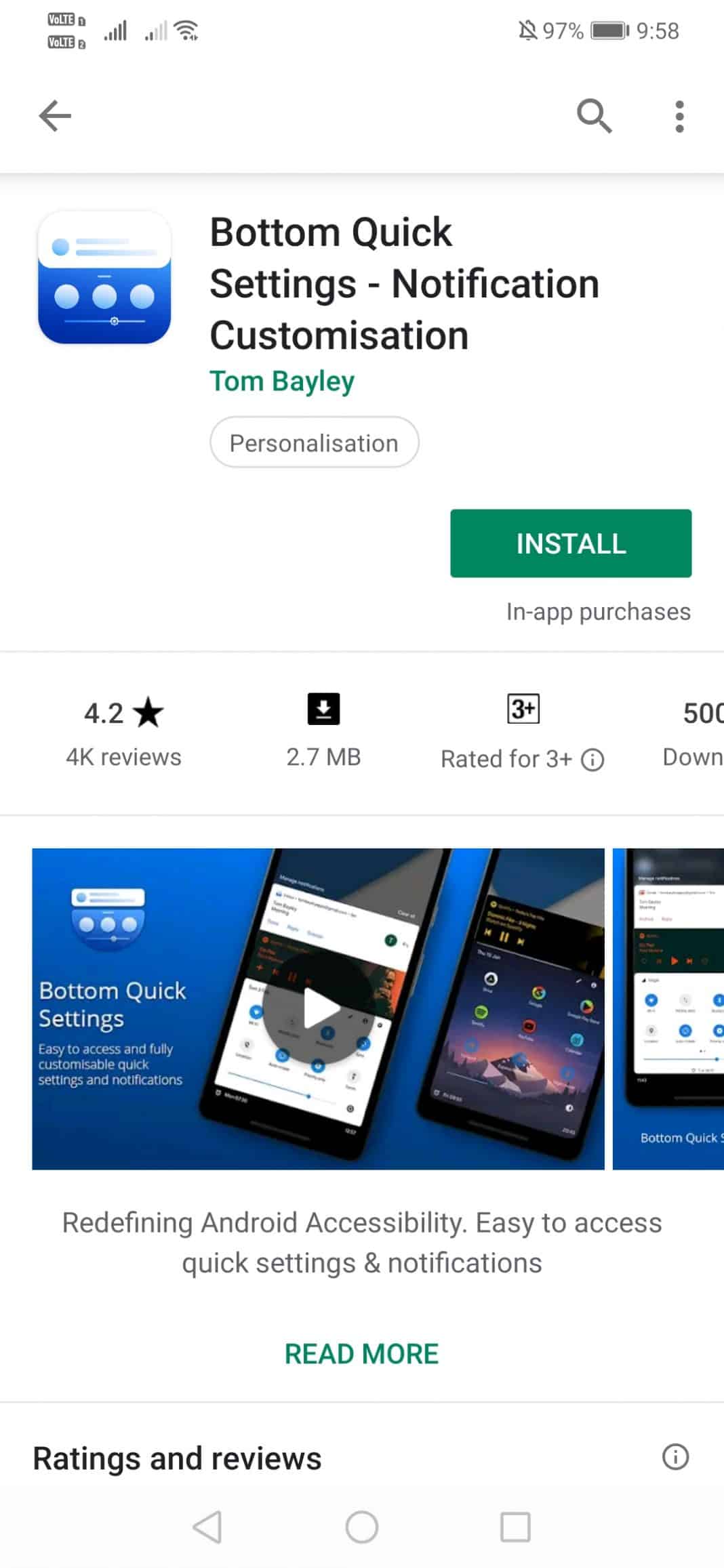A detailed, cleaned-up caption for the described image:

---

The screenshot shows a mobile phone display featuring several status indicators at the top, including "VoLTE 1" and "VoLTE 2" bars, a Wi-Fi signal bar, and a 97% battery icon. The notifications are off, and the time is displayed as 9:58 AM. Below this top section, there are navigational icons—a back arrow, a search bar, and three dots indicating additional settings.

The main part of the screenshot is from an app listing in the Google Play Store. The background is white, and the featured app is "Bottom Quick Settings - Notification Customization" by developer Tom Bailey. The app's logo is displayed, featuring a blue background with a white icon. Directly below the logo is a green "Install" button, with a note indicating that in-app purchases are available.

Further down, the app’s rating is shown as 4.2, along with additional details and images of the application to give prospective users more information.

---